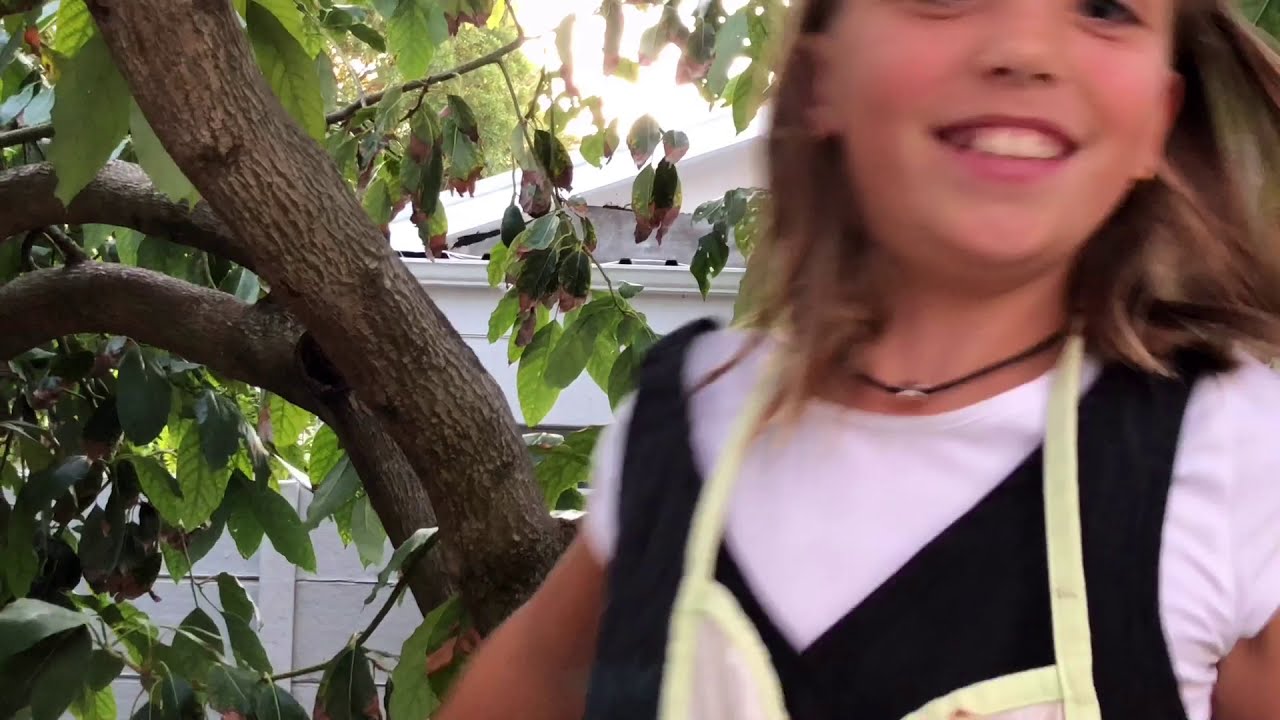The image depicts a slightly blurry close-up of a smiling young girl, likely a preteen, who is Caucasian with light, blonde hair that brushes her shoulders. She is situated mostly to the right within the frame. Her outfit is distinctive, consisting of a short-sleeved white shirt, a black vest or dress, and a yellow apron or smock layered on top. A black necklace featuring a bee adorns her neck. The background reveals a white house and a tree with green leaves that extend towards the picture's top left edge. The lighting suggests a gray or bright sky, adding a natural light to the scene. Her smile and the casual, layered attire, which some interpret as a cooking outfit, hint that she's enjoying a pleasant outdoor activity, possibly in a front yard setting.